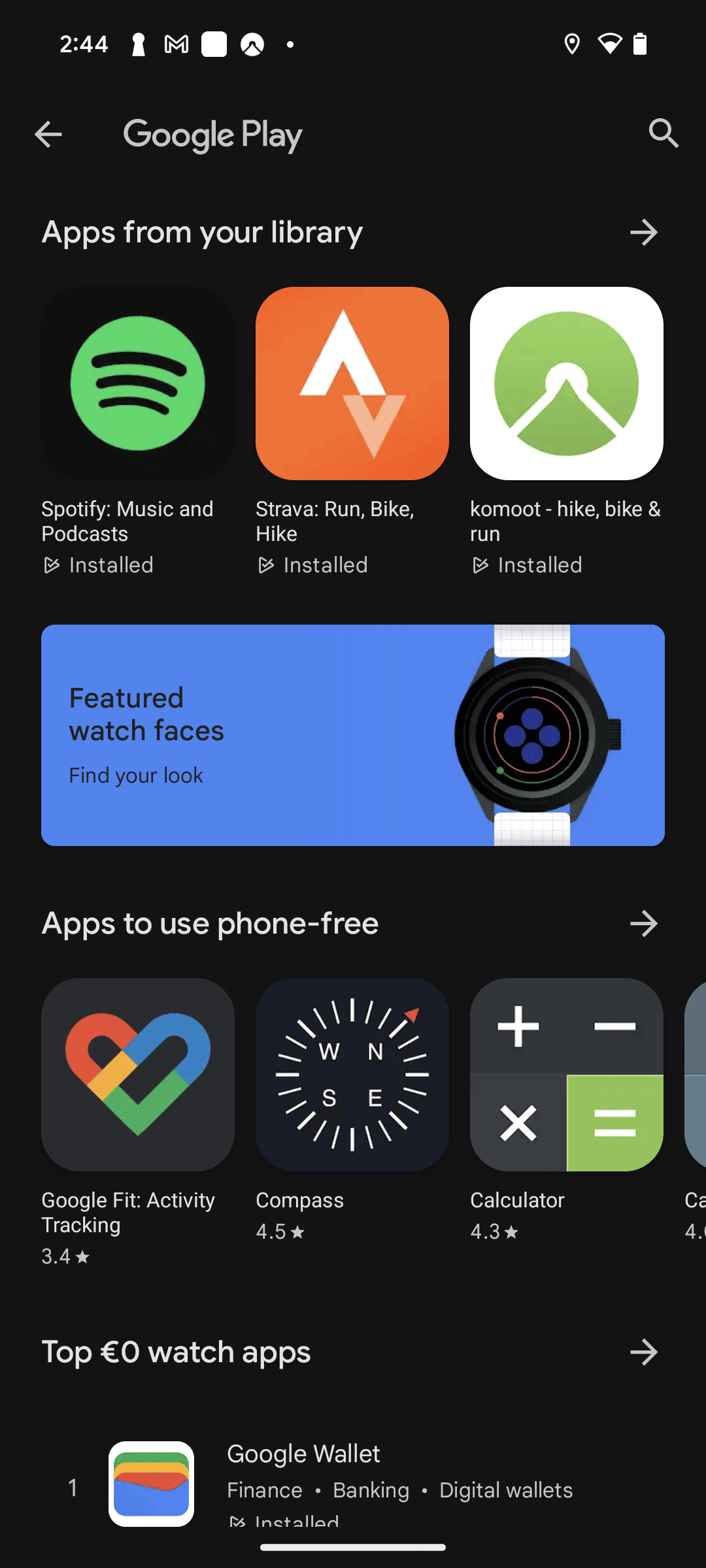The image displays a detailed view of a smartphone screen showcasing various apps and functional icons. At the top left corner, the time is prominently displayed as 2:44, accompanied by several icons, including a lock keyhole, a letter "M," and a mountain peak symbol. On the right-hand side next to these, Wi-Fi signal strength and the battery indicator are clearly visible.

Just below this row, "Google Play" is displayed on the left-hand side, while a search icon is situated on the right. Beneath this section, there is a heading labeled "Apps from your library." The first visible app icon on the left is Spotify, followed by Strava, and then Komoot, with all three apps indicated as installed.

Below these, a blue panel occupies a section of the screen, with an image of a watch on the right. The left-hand side of this panel features the text "Featured Watch Faces" in black lettering, along with the phrase "Find your look."

Underneath the blue panel is another segment titled "Apps to use phone free." This section includes several app icons such as Google Fit, Compass, Calculator, and another potentially different calculator app with a truncated name that isn't fully visible.

Finally, the image shows a heading for "Top Dollar Watch Apps," with Google Wallet listed underneath, signifying it as an app used for financial transactions.